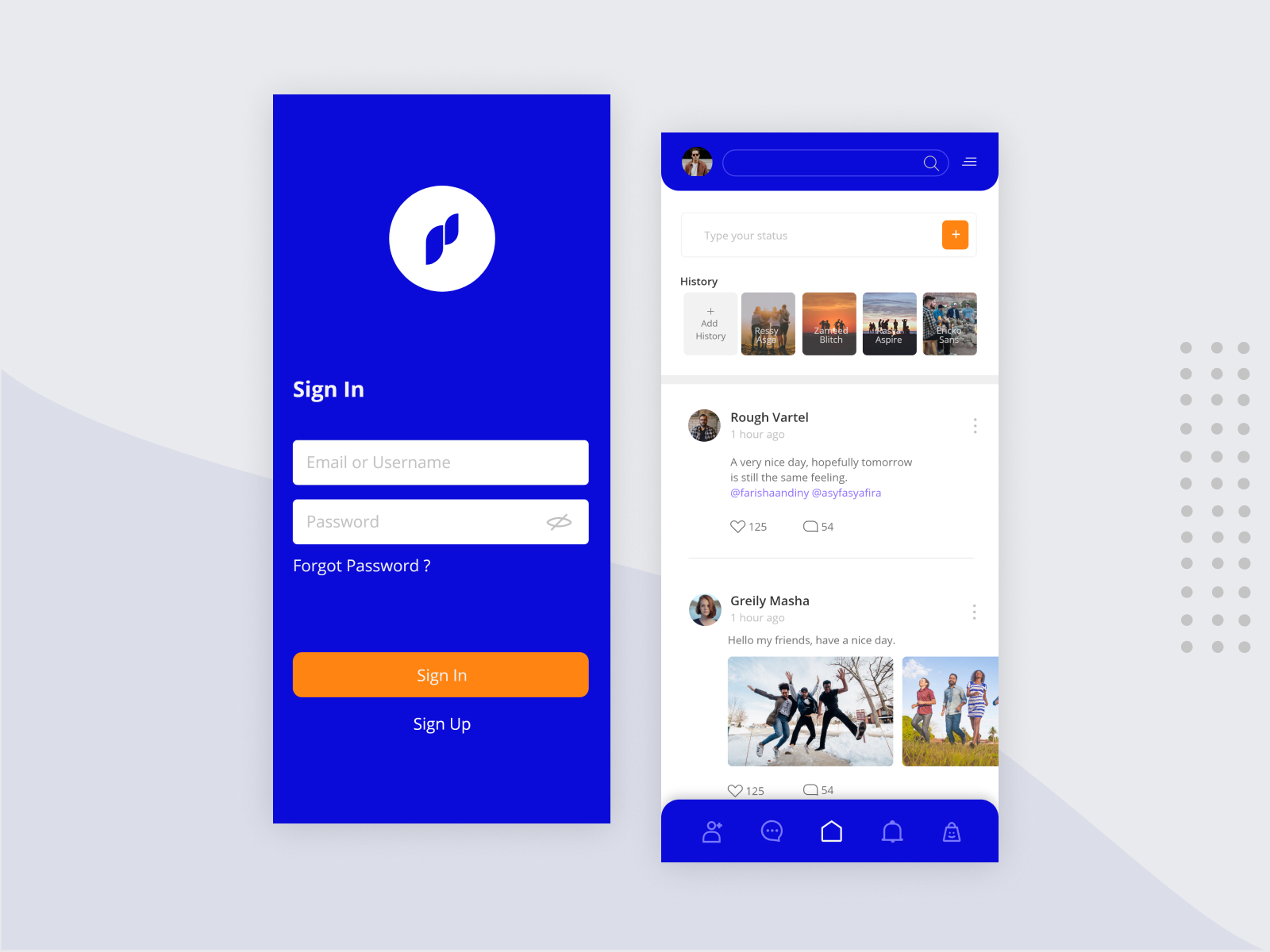This image depicts two smartphone screens placed side by side, set against a background divided diagonally into two shades of gray. The upper area is a lighter gray, transitioning into a darker gray at the lower left corner. From the middle to the right edge, three vertical rows of gray circles run parallel to each other.

The left smartphone screen displays a royal blue rectangular box with a circle icon at the top, featuring blue lines. Below it, the screen prompts the user to sign in with an email or username and password. It also provides options for "Forgot Password," an orange "Sign In" button, and a blue "Sign Up" link.

The right smartphone screen appears to show a messaging or social media interface. It includes a section for conversation history and a text box for typing messages, accompanied by an orange plus sign. Near the bottom of this screen, there are a couple of images displayed.